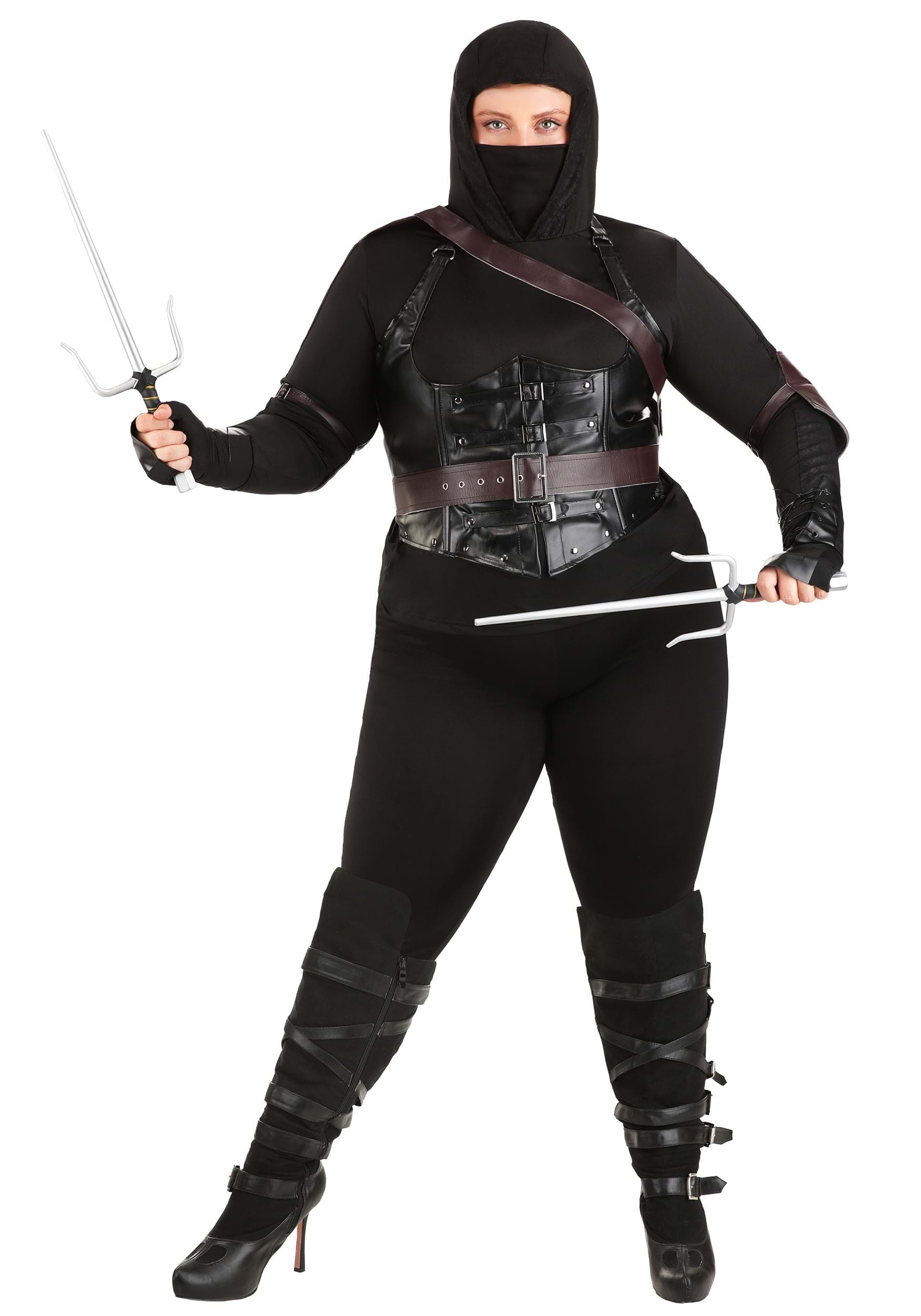The image features a white-skinned woman dressed in an elaborate black ninja costume, set against an all-white background. Her attire includes a skin-tight black bodysuit that covers most of her body, with a black mask and hood revealing only her eyes, eyebrows, and part of her forehead. She wears a black corset over her midsection, accentuated by a brown leather belt that extends over her shoulders and chest. Complementing her outfit are black high-heeled boots adorned with straps that wrap around her calves and shins. She holds two distinctive silver-gray daggers, each with a central long point flanked by two shorter spikes. Her fingers are partially exposed, while the rest of her hands are covered by gloves and brown leather elbow pads. She stands in an aggressive or attacking stance, staring directly at the viewer, exuding an aura of stealth and readiness.